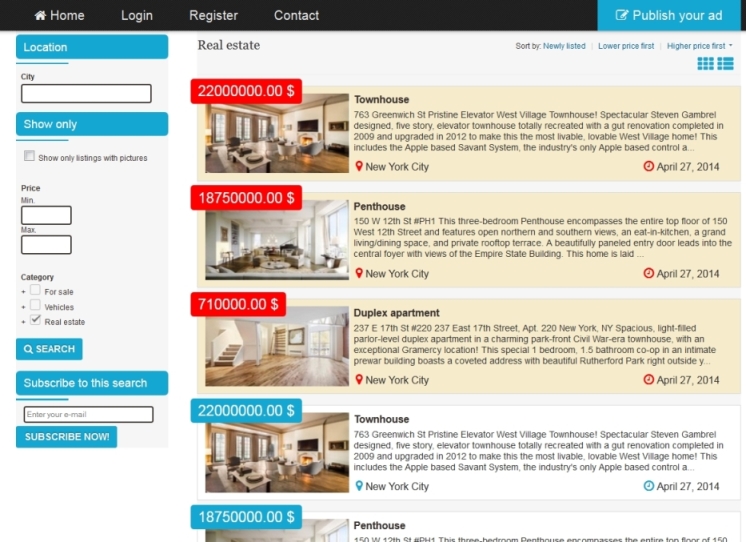**Screenshot of a Real Estate Web Page in Detail:**

The screenshot showcases a real estate website, although it is cropped to focus on the essential elements. At the very top, a black horizontal navigation bar spans the width of the page, featuring the following menu options from left to right: "Home," "Login," "Register," and "Contact." To the far right of this bar, a blue rectangle with white font invites users to "Publish Your Ad."

Directly below the navigation bar, on the left side, lies a vertical sidebar set against a gray background. The top section of this sidebar contains blue rectangular buttons, starting with a "Location" label. Beneath it, there's a text box designated for inputting a city name. Following this, another blue rectangle sports the label "Show Only," with an option immediately below for users to check a box to filter listings to only those with pictures.

Further down, the sidebar provides options to input a price range with fields for "Minimum" and "Maximum" amounts. Additional search filters are available under the "Category" label to refine the search criteria even more. At the bottom of this comprehensive search filter section, there is a prominent blue search button.

Continuing downward, the sidebar features a larger blue rectangle prompting users to "Subscribe to the Search." Below this prompt, there's an input field labeled "Enter your email," along with a final blue rectangle that says "Subscribe Now." 

On the right side of the page, the main content section begins with a heading labeled "Real Estate." Beneath this heading, a series of property listings are displayed in a vertical format. Each listing consists of a few key elements: the price is prominently displayed in the top left corner above a thumbnail image of the property, which is also positioned on the left. To the right of each thumbnail, a brief property description provides details about the listing. Finally, in the bottom right corner of each listing, the date the listing was posted is noted.

This organized layout allows users to seamlessly search through various real estate options using a range of filters and subscribe for updates according to their specified criteria.